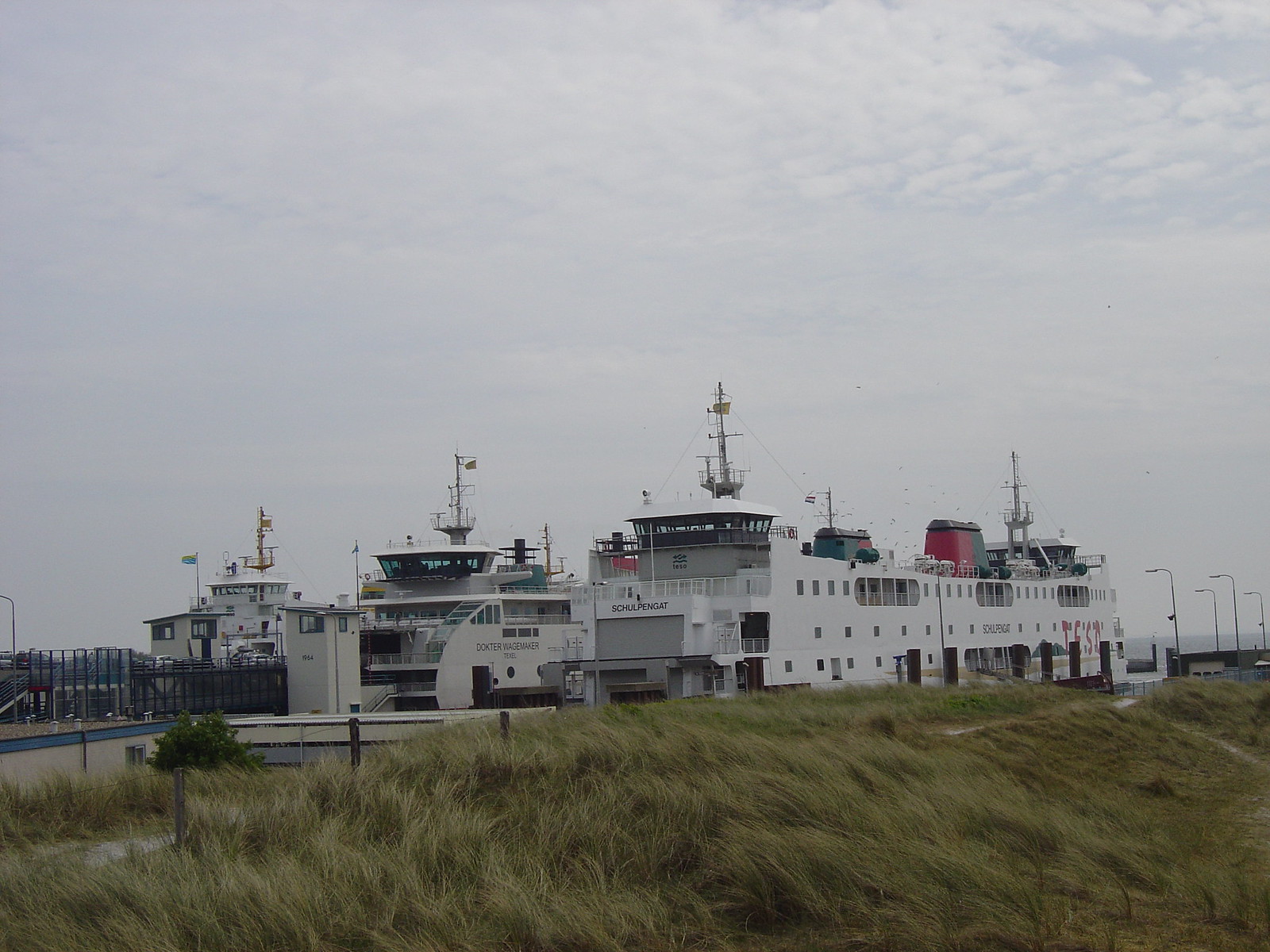The image depicts three large, white cruise ships, two of which are situated in a canal-like waterway that resembles the Panama Canal, while the third ship is positioned slightly further back. Each ship features approximately 30 rooms spread across three floors, indicating a high capacity for passengers. A prominent feature on these vessels is the captain's house, encased in glass, positioned at the front of each ship. Additionally, the ships are equipped with various towers, smokestacks in gray and red, and observatory-like structures.

In the foreground, a field of long, thin grass bends with the wind, suggesting strong air currents. This grassy area precedes a slightly elevated hill that obscures direct water visibility. Despite the lack of visible water near the grassland, the canal’s context and structure are evident behind this foreground. Telephone poles and light posts punctuate the hazy, cloudy background, along with a few faintly visible trees.

On the closer ship, a large gray area and a red feature are noticeable on the roof. Smaller details like the garage-type door on the front and numerous small windows lining the side add complexity to the scene. Names and writing adorn the sides of these ships, although the text is too distant and not in English, making it indecipherable. Also scattered in the background are some metal fencing and poles, hinting at further infrastructure related to the canal. The overall atmosphere feels industrious and somewhat concealed by the overcast sky, emphasizing the formidable size and preparedness of these maritime giants.